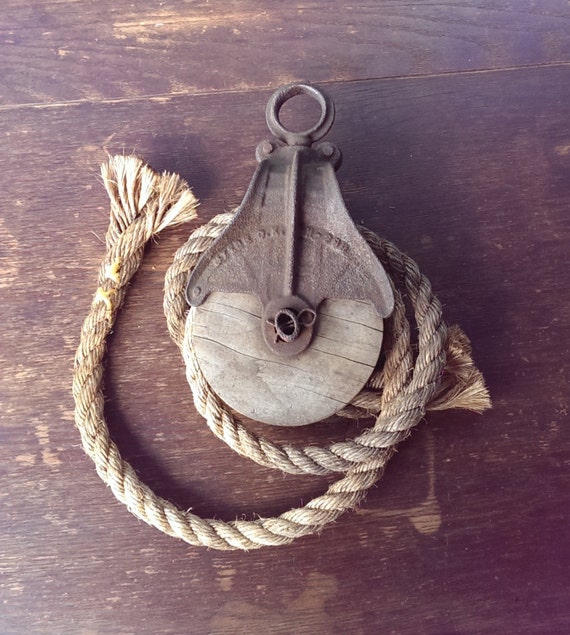This detailed color photo showcases a close-up overhead view of a vintage pulley system, featuring a rustic aesthetic with clearly visible wear and tear. The pulley, composed of wood and iron, exhibits a charming aged patina. At the top of the pulley is a large, metal circular hook or loop, designed for hanging. Below, a thick, weathered rope, with a faded white hue, is loosely coiled around the wooden spool of the apparatus. The rope appears to be frayed on both ends, with one end laying to the left side of the pulley. The entire pulley system is positioned flat on a dark, richly textured wooden table that bears the marks of time, including nicks, cracks, and water stains. This setting further enhances the antique and decorative nature of the pulley, suggesting it could be a distinctive piece for home decor.